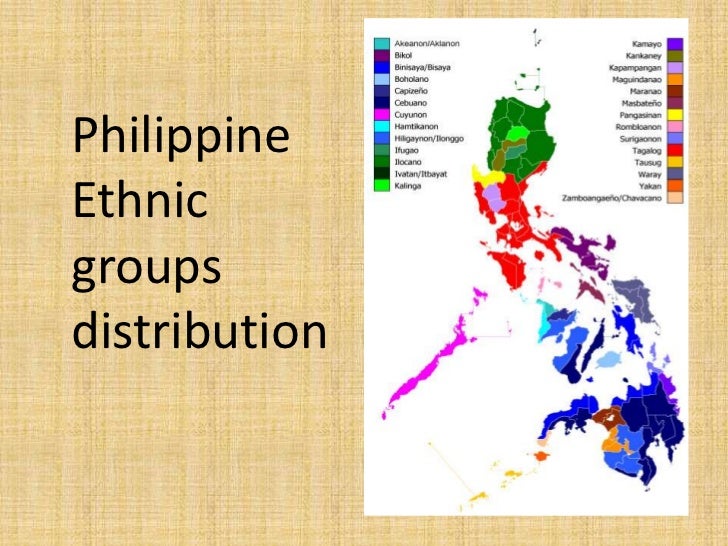The image displays a detailed map of the Philippines, highlighting the distribution of various ethnic groups through a diverse color scheme. The map transitions through multiple colors: starting with green at the top, shifting to yellow, red, purple, magenta, darker purple, dark dual gray, blue, dark navy blue, more purple, and other distinct hues such as orange, pink, peach, turquoise, and brown. Accompanying the map is a key that assigns each color to a specific ethnic group, with labels like "Cameo," "Rambangan," "Kayunan," "Imbankyo," and "Biko," among others, some of which are in a language not easily recognizable. 

The map itself is set against a white background, and the entire slide is framed with a light yellowish-beige, textured backdrop resembling a checkered or plaid pattern, akin to a burlap sack. The map is contained within a white rectangular cutout on the right side of the slide. The title, "Philippine Ethnic Groups Distribution," is prominently displayed in black text, providing a clear understanding of the map’s purpose.